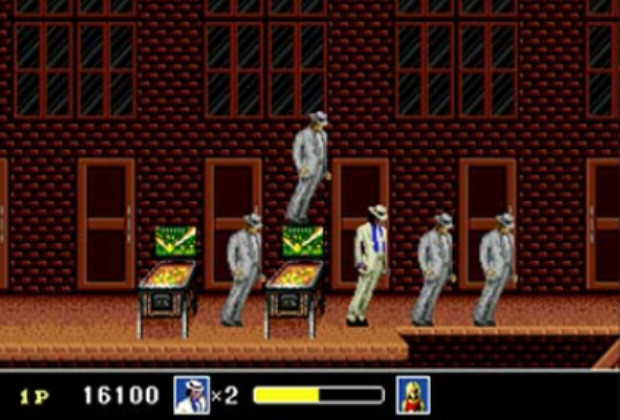The screenshot depicts a scene from a video game inspired by Michael Jackson's "Smooth Criminal." The background showcases a red brick wall adorned with multiple orange and brown doors, resembling an apartment building with rows of four-paned windows above them. The stage, patterned in brown and orange, features two forward-facing pinball machines. In the center, Michael Jackson stands out in a goldish-yellow suit with a blue lapel, and a cream hat with a blue band, different from the other four characters who all don white suits and white hats. These characters, along with Jackson, are leaning sharply to the right, seemingly defying gravity in a plank-like pose. One character stands between the pinball machines, while another intriguingly balances on the back of a pinball machine. The bottom of the screen displays game details: "1P" followed by the score "16100" in white, an icon of a character in a white suit with a count of lives left (two), and a half-yellow, half-black horizontal bar. Additionally, there's a square icon showing a person in a red top with possibly blond hair, though the details are indistinct.